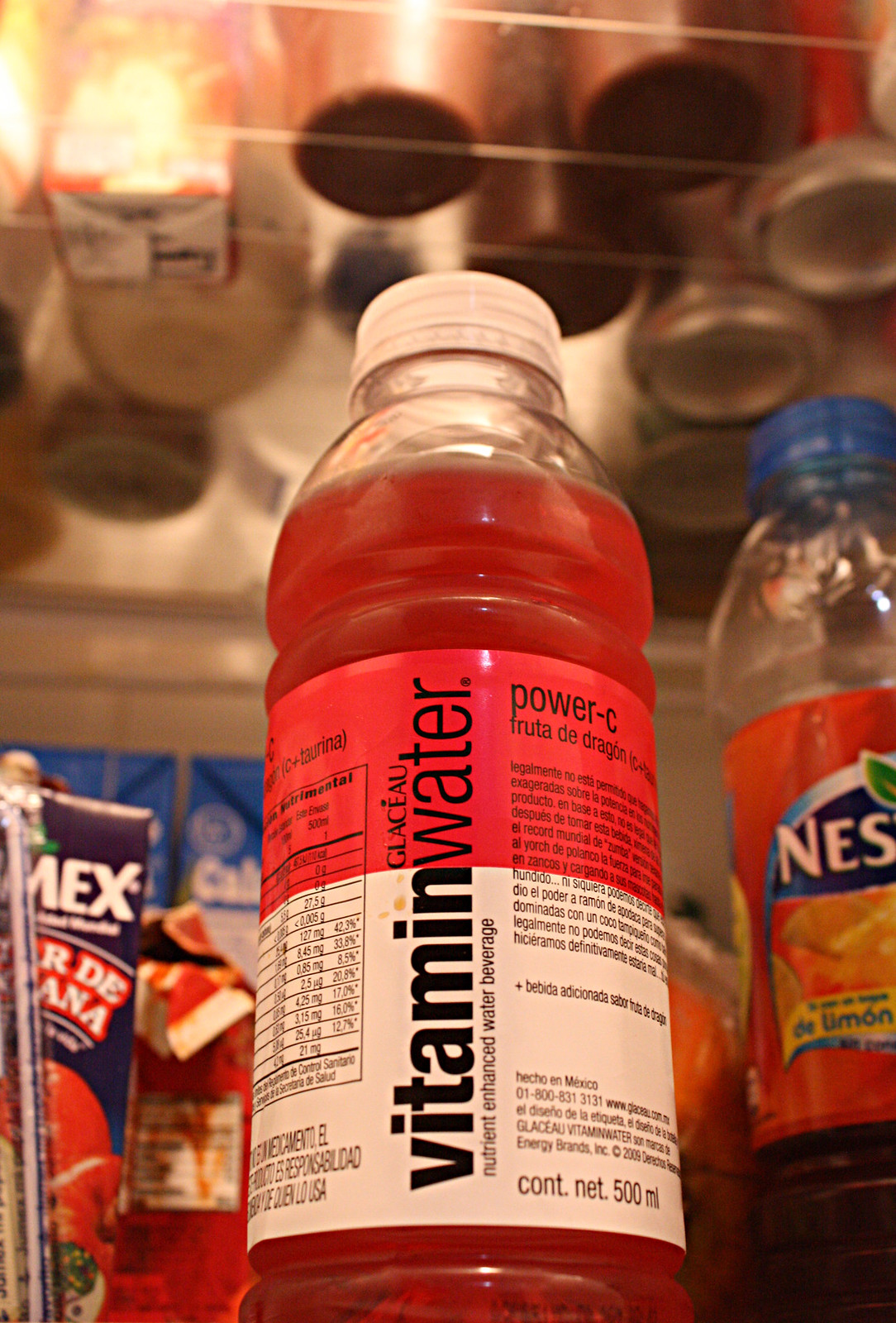This photograph showcases a bottle of Glaceau Vitamin Water lying on its side, with the vibrant red beverage visible through the transparent plastic. The label incorporates a mix of white and light red hues, veering towards orange, with various writings and nutrition information, although the text is not fully legible. The bottle has a white cap. Adjacent to this bottle is another, likely a Nes-T brand, visible through the partially obscured "N-E-S" on its label. This bottle is clear, potentially containing a small amount of liquid at the bottom and is topped with a blue cap. To the left of these bottles, there are several packages, displaying a partial text, "M-E-X," possibly denoting used food packaging. In the background, an assortment of pots and pans is visible, adding context to the kitchen setting of the scene.